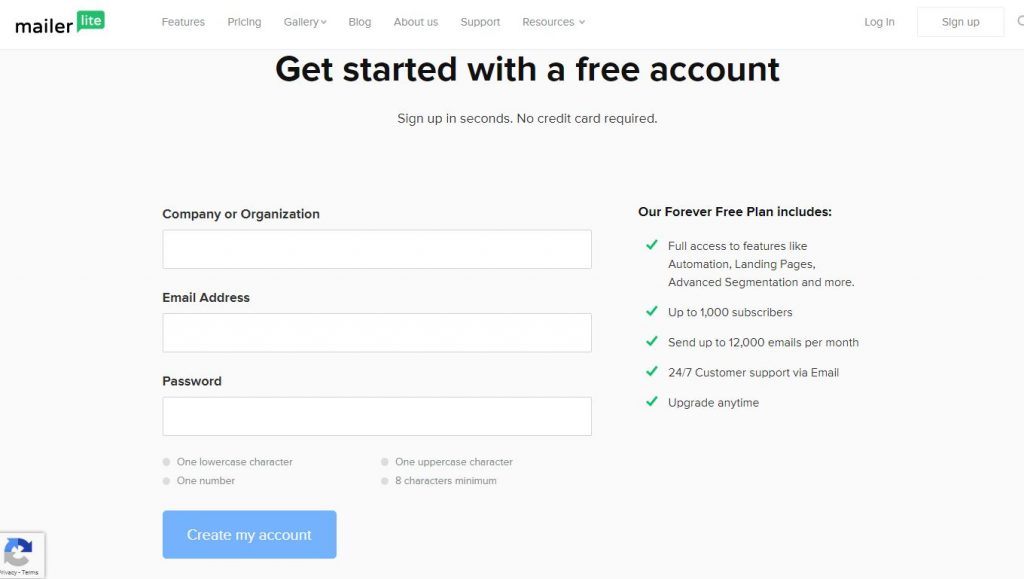The image is a horizontal rectangle, with a crisp white background on the left side, featuring the word "mailer" in all lowercase, bolded black font. Adjacent to this is a small green bubble containing the word "lite" in lowercase, white font. 

Across the top, next to "mailer," there are light gray menu headers: "Features," "Pricing," "Gallery" (with a small downward arrow icon), "Blog," "About Us," "Support," and "Resources" (with another downward arrow icon). To the far right, there are rectangular buttons for "Log In" and "Sign Up" with a horizontal layout.

Below this is an off-white section. Centered along the top edge in large bold black font is the phrase "Get started with a free account." Directly underneath, in regular black font, it reads, "Sign up in seconds, no credit card required."

The content is divided into two columns. The left column contains fields for signing up, with instructions in black font:
- "Company or Organization" followed by a horizontal rectangular white input box outlined in gray.
- "Email Address" followed by a similar white box.
- "Password" followed by another white box, along with some password rules beneath it.

At the bottom of the left column is a light blue rectangular button with white font that says, "Create My Account."

The right column has a list in black font with a bold header that states, "Our forever free plan includes:" Each feature is prefaced by a small green checkmark and includes:
- Full access to features like automation, landing pages, advanced segmentation, and more
- Up to 1,000 subscribers
- Send up to 12,000 emails per month
- 24/7 customer support via email
- Upgrade anytime

At the very bottom, emphasized in blue is another call-to-action button that reads, "Create My Account" in white font.